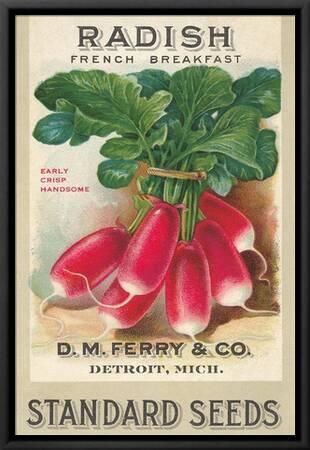This image depicts a vintage vegetable poster, likely from the 1930s or 1940s, framed with a thin black plastic border. Measuring approximately three inches high by two inches wide, the poster features a tan background with watercolor markings that subtly bleed into the image. At the top of the poster, in bold gray print with a shadow outline, the word "Radish" is prominently displayed. Beneath it, "French Breakfast" is written, and below that, an artistic rendering of a bunch of six radishes, bound together with a tan rubber band, is illustrated. These radishes are characterized by their raspberry-red color fading to white at the tips, complete with green stems and leaves. Adjacent to the radishes, in bold red font, the text reads "Early Crisp Pansum." At the bottom of the poster, in dark gray print with a light gray shadow, it states "DM Ferry and Co. Detroit Michigan Standard Seeds."